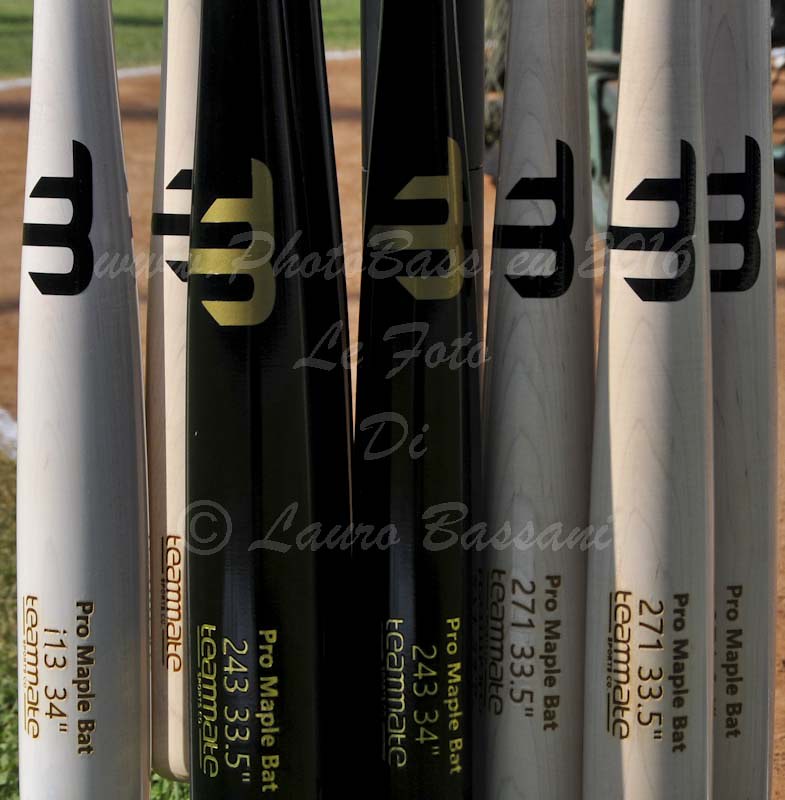This square photograph, watermarked by Bodo Bass in 2016 with additional copyright by Laura Bassani, offers a detailed, close-up view of eight vertically positioned baseball bats. The bats, positioned on a baseball field featuring chalk lines and reddish dirt against a grassy backdrop, partly obscure their handles as they taper away from view. Seven of these bats showcase an 'M'-shaped logo, with the captions "Pro Maple Bat," "271," and "33.5 inches" followed by an underlined "Teammate" inscribed near their thicker ends. The bats vary in color, with three pale wooden bats adorned with a black 'M' logo, two black bats marked with a golden 'M' logo, and two white bats also featuring a black 'M' logo. Some bats exhibit minor burn marks, adding to their distinct appearance.